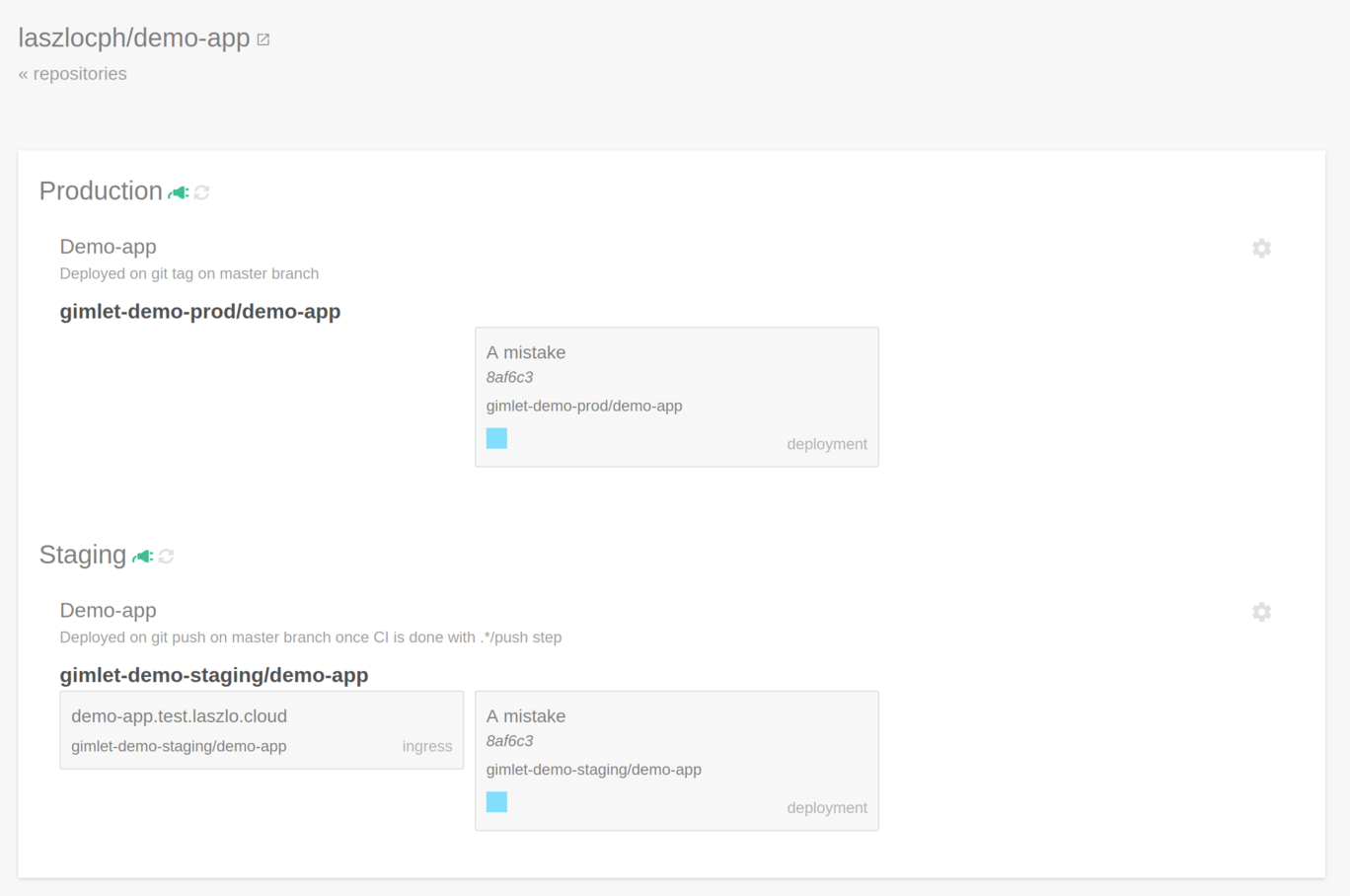Screenshot of an application interface. In the upper left-hand corner, the text "LASZLOC-PH\demo-app" is displayed. Below that, in a large white section labeled "Production," it says "demo app deployed on git tag on master branch," followed by "gimlet-demo-prod\demo-app." Under the "Production" section, there's another menu labeled "Staging." Beneath this, it states that the demo app is "deployed on git push on master branch once CL is done with *\push step." This seems to be an interface for managing code deployments and stages in a software development environment.